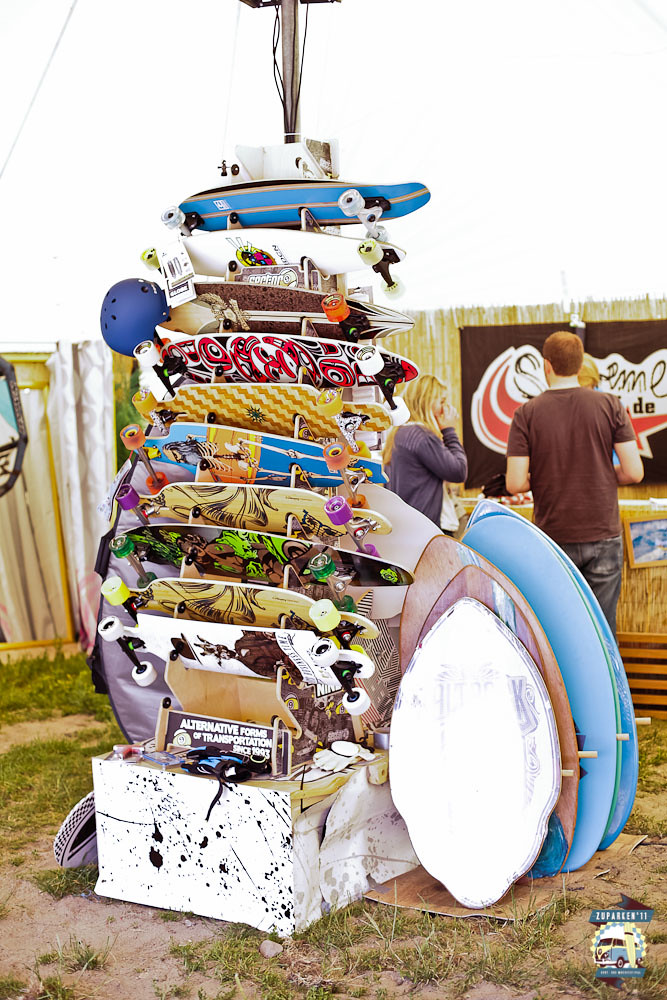The image is a vertical rectangle photograph taken outdoors during the day, evident by the light gray sky above. The bottom surface is a mix of light brown dirt and grass, bordered in the background by a wooden fence with various signs, possibly indicating an outdoor store. Central in the photo is a vibrant display of skateboards stacked on a tall white rack with a black splatter pattern. The rack is topped with numerous colorful skateboards, each featuring unique designs—blue, white, brown, white with a red tribal design, yellow zigzag pattern, blue with a skeleton, yellow and black, and brown and green. Just below the skateboards lie skateboarding tools such as fingerless gloves and a bumper sticker reading "alternative forms of transportation since 1993."

To the right of the skateboard rack, there are skimboards in white, blue, and brown, neatly arranged on a white display shelf. Hanging off the left side of the skateboard rack is a blue helmet. Nearby, a white man with short red hair in a red short-sleeve shirt and jeans stands next to a white woman with blonde hair in a brown sweater. These two individuals, with their backs towards the camera, seem to be engaged in examining a poster or a register, adding a human element to the scene. The image captures a dynamic and colorful outdoor setting.